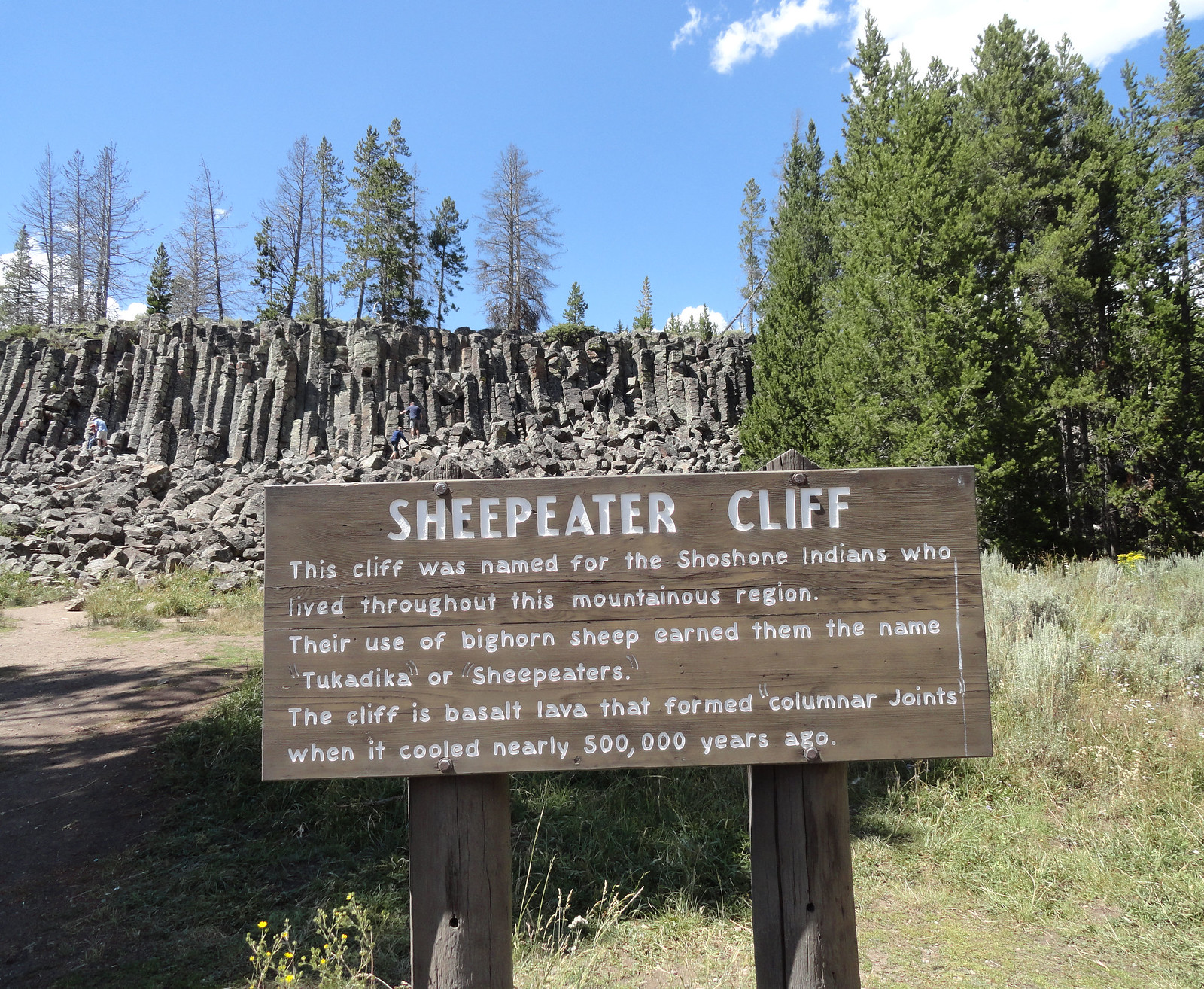The image captures an outdoor scene dominated by Sheep Eater Cliff. In the foreground, a wooden sign mounted on two posts reads, "Sheep Eater Cliff." The sign explains that this cliff was named after the Shoshone Indians, whose use of bighorn sheep earned them the name Tukadika, or Sheep Eaters. The cliff itself is composed of basalt lava that formed columnar joints when it cooled nearly 500,000 years ago. Behind the sign, the rugged cliff showcases its distinct columnar structure. A blue sky with a few clouds forms the backdrop, highlighting the daytime setting. The area is dotted with pine trees, some of which are devoid of needles, while others are lush and green. At the base of the cliff, rocky terrain is visible, with a few people walking or climbing the rocks. Among the grassy field are patches of weeds with somewhat yellow flowers, adding a touch of color to the natural landscape.